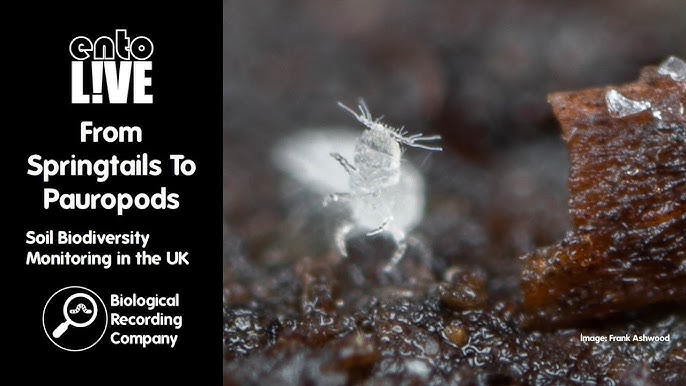The photograph depicts a detailed, close-up view of a transparent, white microscopic insect-like creature, possibly a springtail or similar arthropod, moving through moist brown soil. The creature, which has an oval-shaped head, a long segmented body, six legs, and antennae, is shown from the front, appearing to rise slightly off the ground as it traverses the terrain. On the right-hand side of the image, the soil is shown in vivid detail, with its moist texture and varying shades of brown. There's a blurry chunk of brown material, possibly wood or a rock, further indicating the natural setting.

On the left side of the image, a vertical black rectangle contains white text reading "EntoLive: From Springtails to Pauropods, Soil Biodiversity Monitoring in the UK." Below this, the logo of the Biological Recording Company is depicted, featuring a white magnifying glass with a small white worm inside it. At the bottom right of the image, the text "Image: Frank Ashwood" identifies the photographer. The overall composition is laid out as a horizontally oriented rectangle, about twice as wide as it is tall.